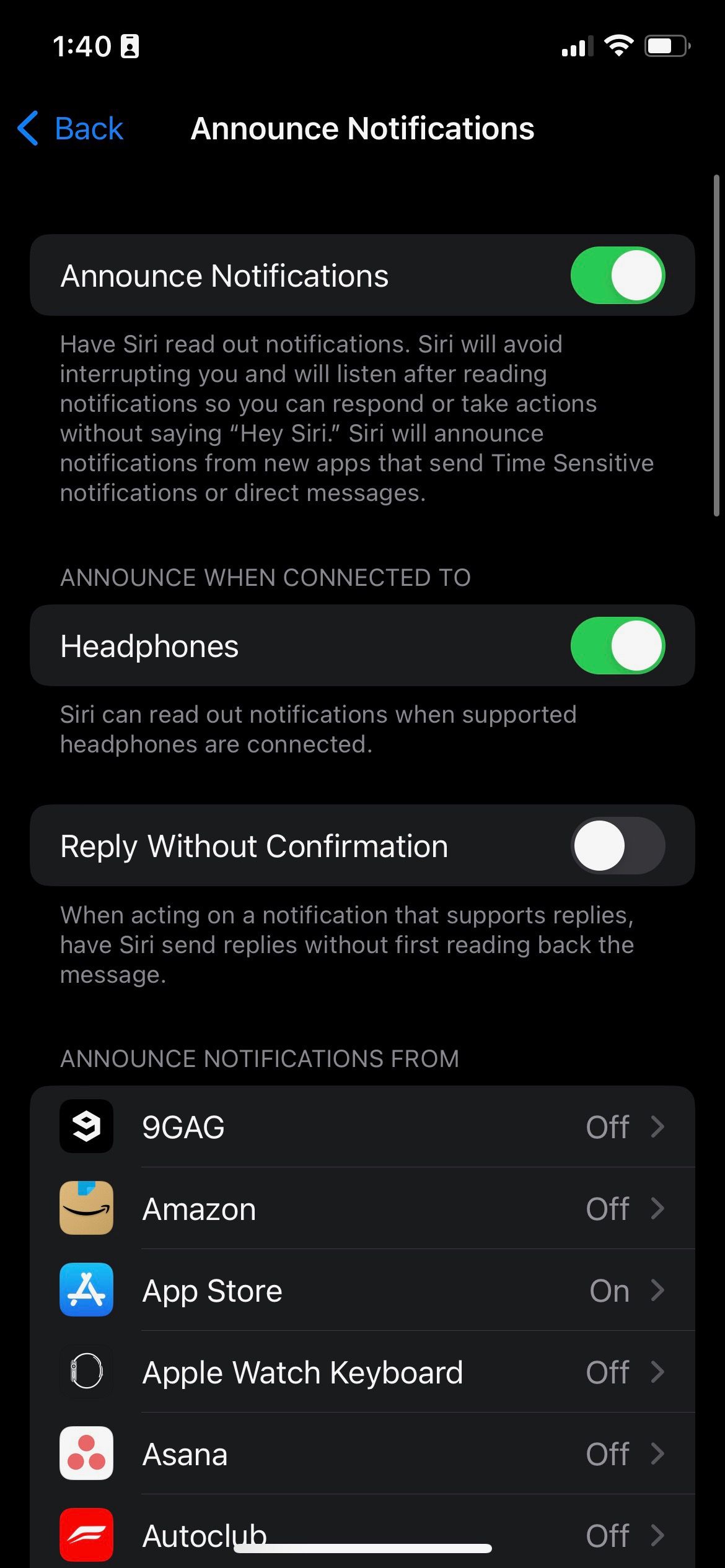Screenshot of a mobile phone display, suggesting a current time of 1:40 PM, indicated by the top menu bar. The status icons include a Wi-Fi signal, data signal, and a battery indicator showing approximately 75% charge remaining. The phone is likely in night or dark mode due to the black background.

At the top of the screen, there is a blue arrow with blue text reading "Back." The main header, "Announce Notifications," is displayed prominently in bold white text. Below it, a description appears in smaller, grayish text: "Have Siri read out notifications. Siri will avoid interrupting you and will listen after reading notifications, so you can respond or take actions without saying, 'Hey Siri.' Siri will announce notifications from new apps that send time-sensitive notifications or direct messages."

A green toggle switch indicates that the "Announce Notifications" feature is enabled. Following this, another setting titled "Announce When Connected to Headphones" is also turned on. The next option, "Reply Without Confirmation," remains disabled with a gray toggle switch. Finally, the section "Announce Notifications From" lists several apps with on/off toggles: 9gag, Amazon, and App Store, indicating selective notification announcements for these apps.